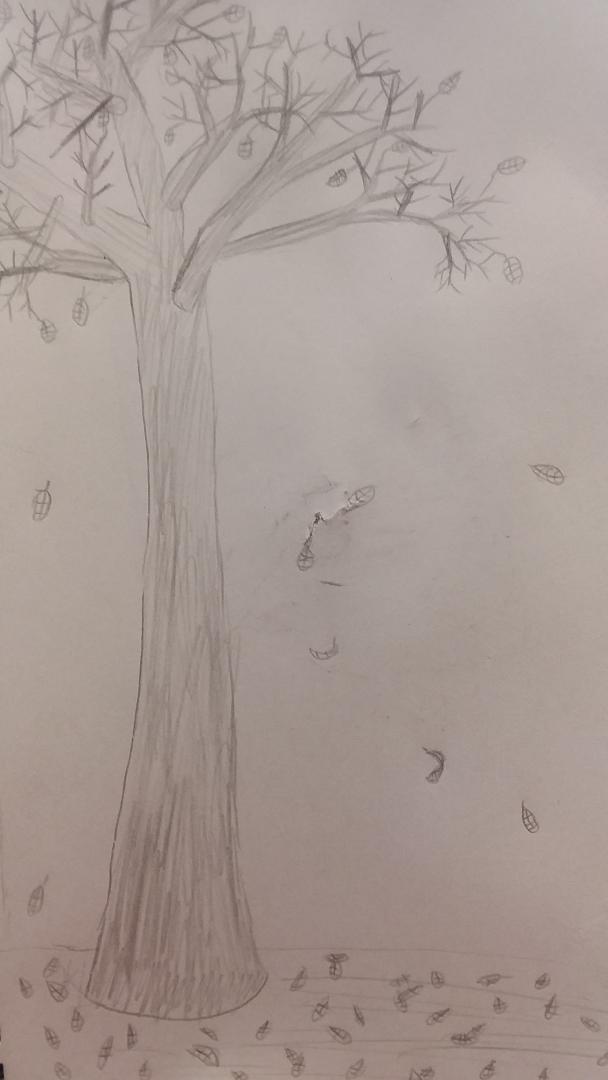This is a simple yet evocative pencil drawing, characteristic of an older child's artistic effort, depicting a tree in the autumn season. The illustration is crafted on a plain white sheet of paper, oriented vertically. Dominating the left side of the composition is a large and tall tree trunk, intricately detailed with multiple Y-shaped branches extending from its top. Scattered sporadically among these branches are a few singular leaves, each attached delicately to its respective branch. In a beautiful display of autumnal transition, some leaves are illustrated in mid-fall, appearing to be gently suspended in the air. A noticeable tear mars the paper, evidence of a moment where the artist erased too vigorously. Accumulating gracefully on the ground below the tree are a number of leaves that have already fallen, adding to the seasonal atmosphere of the scene. The entire depiction is rendered in varying shades of gray, utilizing the simplicity and depth of a lead pencil to bring the scene to life.